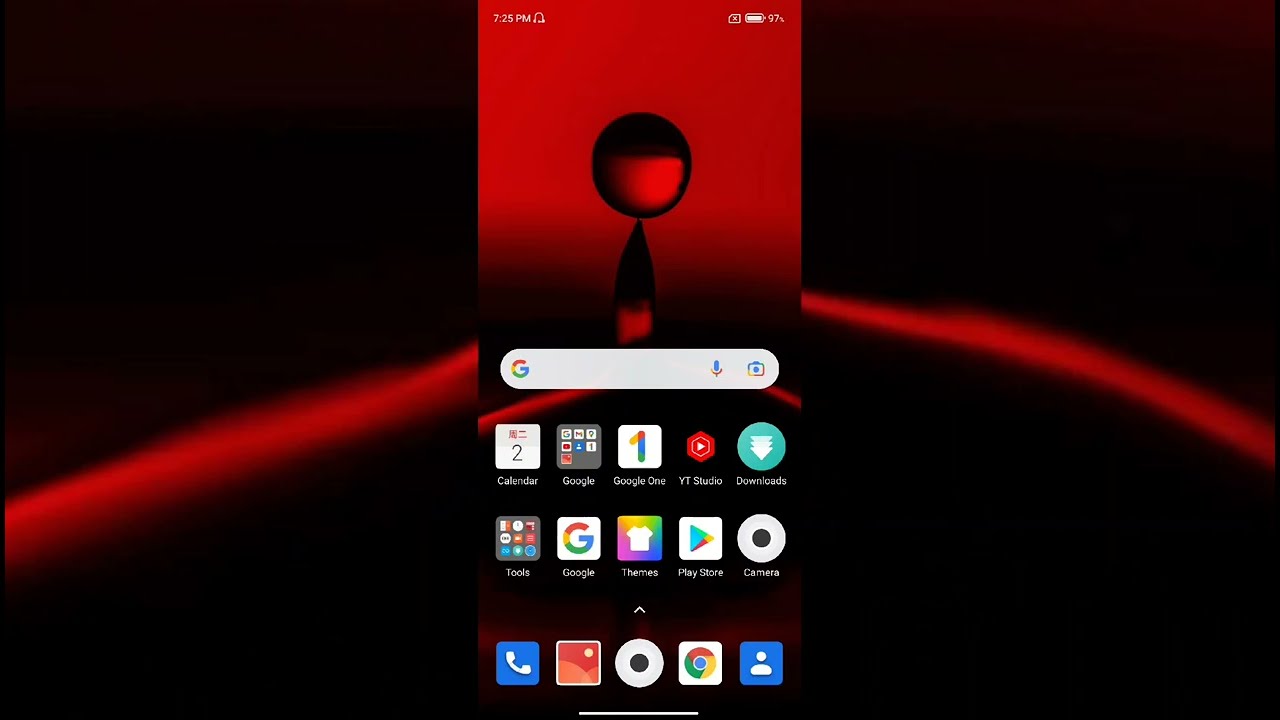The image is a screenshot of a smartphone home page. The background features a striking design with red and black hues, dominated by a central figure resembling a ball perched on a pointed column, split into red and black halves. At the top of the screen, the small time display reads 7:25 p.m., and the battery shows a 93% charge. Central to the display is a prominent white search bar with the Google 'G' logo and a microphone icon. Below this, the home screen showcases commonly used apps like Calendar, Google, Play Store, and Gmail. The bottom section includes navigation icons such as a blue and white phone, a center home button, and another Google button, accompanied by a blue-marked person icon. The arrangement and typical Android interface suggest this is likely an Android device.